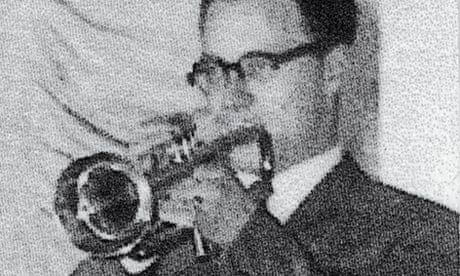In this very grainy, black and white photograph, a faded, cropped portrait of a man from the shoulders up is captured playing a brass instrument, possibly a trombone. He faces slightly to the left, featuring distinct black-rimmed oval glasses and dark hair receding with a high forehead. Although his facial features are not clearly defined due to the low resolution, he appears to be a Caucasian male with a round face, partially bald, and dark hair at the back of his head. The background, seemingly a folded sheet, casts some subtle shadows. Dressed formally in a black suit, white shirt, and black tie, he has a ring on his finger, barely discernible. The instrument he plays, although uncertain if it's a trombone or a trumpet, is dark at the large opening, extending towards the viewer.